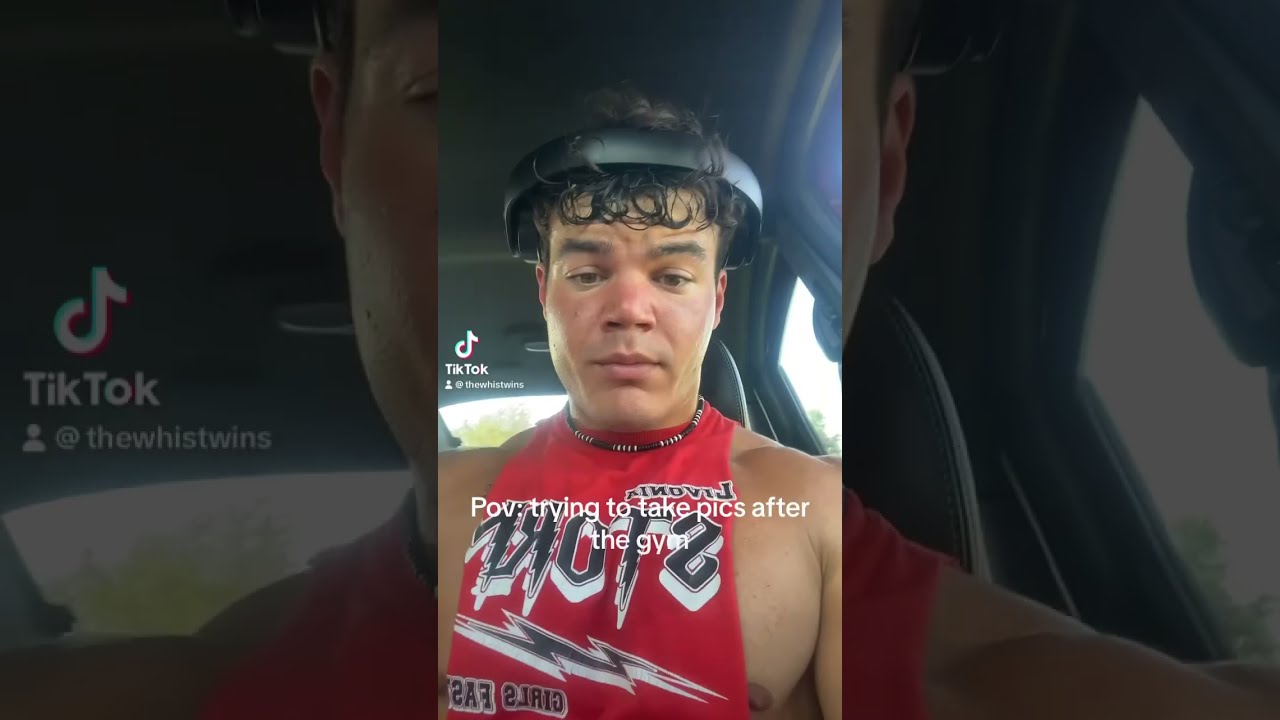The image is a snapshot from a TikTok video featuring a young, muscular, Caucasian man in his early 30s. He is sitting inside a car with a gray interior, and you can see daylight outside. The man appears to have just finished a workout, as he's sweaty and his short black hair is wet and matted. He is clean-shaven and is wearing headphones that are positioned above his ears, resting on his hair.

He is dressed in a red, sleeveless, cutoff T-shirt that has a logo in a 3D lightning bolt style font which seems to spell out "STO..." or "STORT." His brown nipple and a necklace with brown and white beads are visible. The shirt has text, possibly reading "girls at FAS...," though it's unclear. 

Overlaying the image is the caption: "POV trying to take pics after the gym." The TikTok logo and the username "The West Twins" are visible on the left side of the image. The image is divided into three vertical sections, with the first and third sections showing a darkened close-up of the central photo.